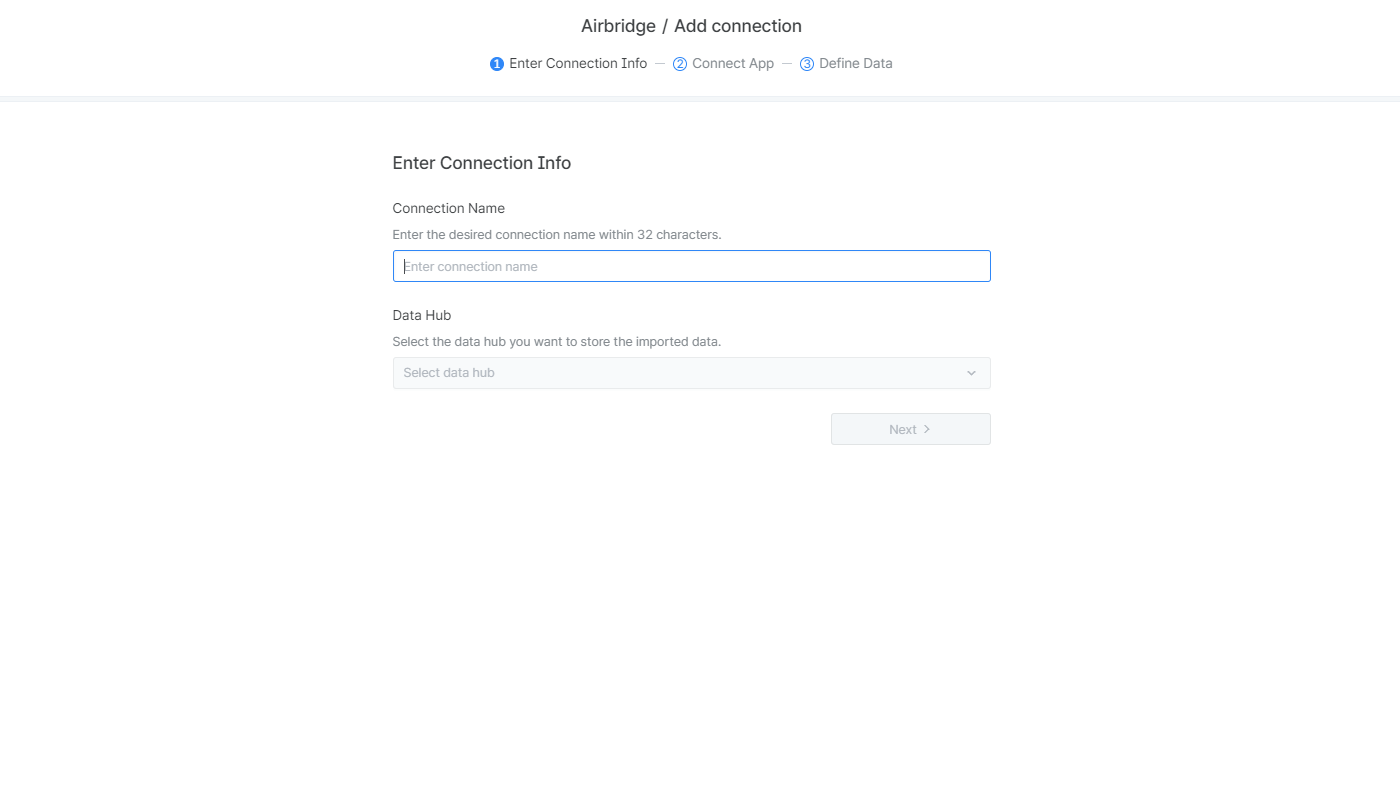This image depicts the "AirBridge Ad Connection" interface. The layout appears center-justified and presents a step-by-step menu for setting up a connection. The first visible item is an option titled "Enter Connection Info," which suggests the current step highlighted by a blue number one. Below this, the subsequent steps are listed: "Connection App" as step two, and "Define Data" as step three. A light gray separator bar is located underneath the step menu, followed by a space. Further down, there is another instance of the "Enter Connection Info" prompt accompanied by a field labeled "Connection Name." A descriptive note specifies users should "Enter the Desired Connection Name within 32 characters," alongside a text input box to complete this information.